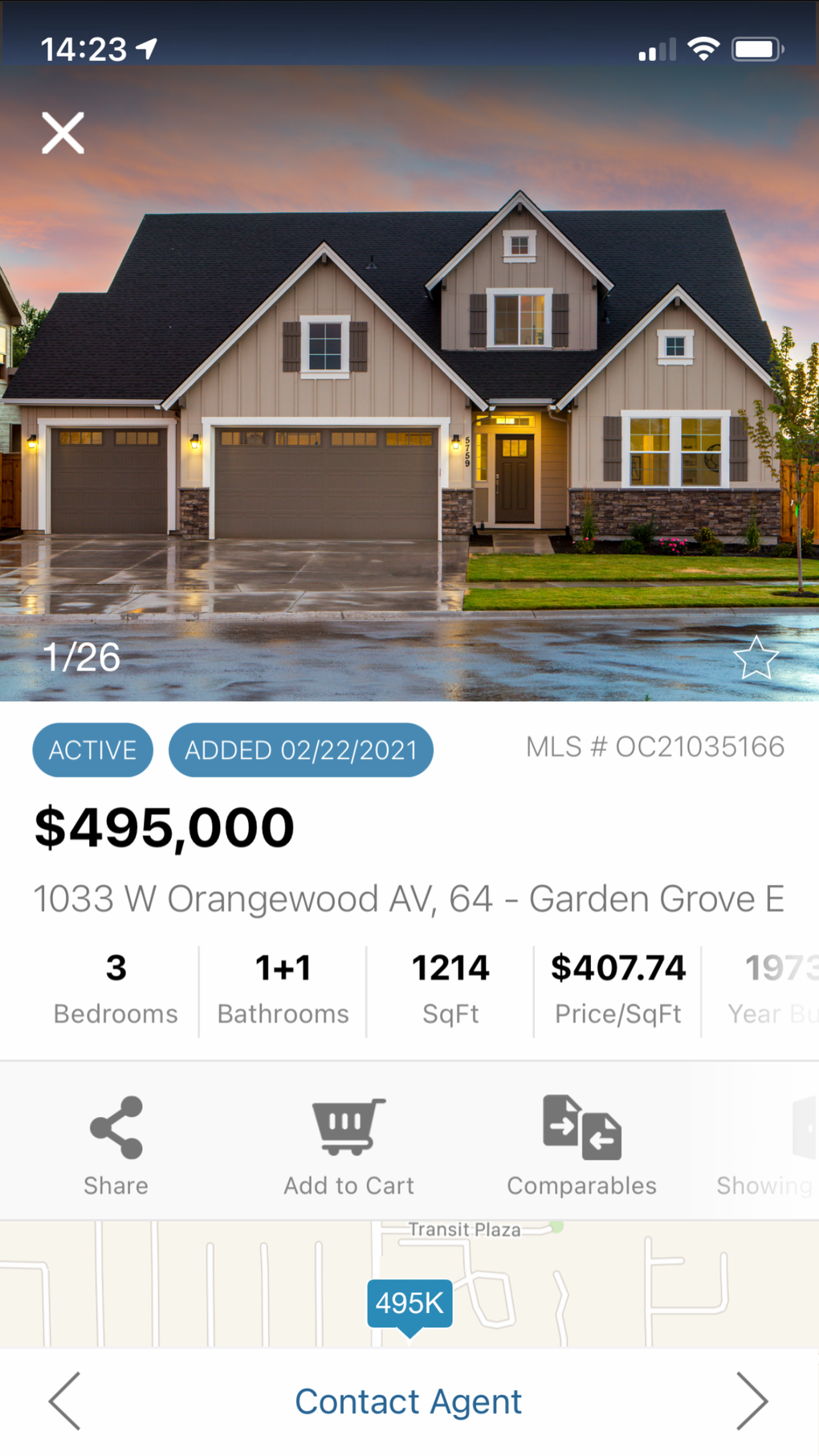This detailed caption describes a screenshot taken from a smartphone, showcasing a real estate listing app. The phone displays various status indicators at the top, including the time (currently 2:23 p.m.), reception details, Wi-Fi status, and battery level.

The screenshot highlights a listing for a home, starting with a photo at dusk, with exterior and interior lights turned on. The house features two garages on the left and an entrance door on the right, accompanied by several windows. The front yard includes a small lawn and a newly planted tree. The screenshot indicates this is the first of 26 available images of the property.

The listing is marked as active and was added on February 22, 2021. Essential details like the Multiple Listing Service (MLS) number, the listing price, the address, and key specifications of the home—such as the number of bedrooms and bathrooms, total square footage, price per square foot, and the age of the property—are all partially visible. Functional options displayed on the screen include buttons to share the listing, add it to a cart, compare it with others, view a map for location details, and contact the real estate agent.